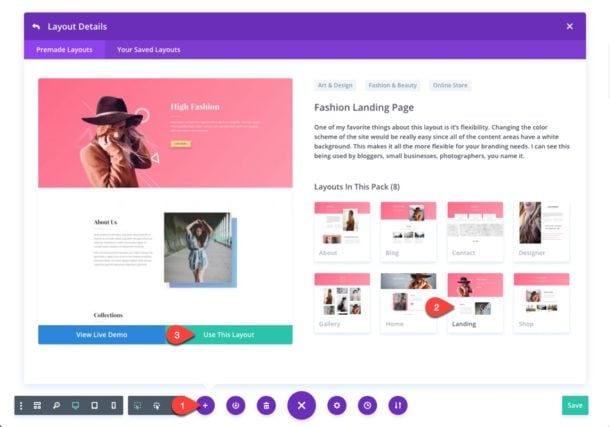This image features a high-fashion landing page design layout showcased in a sophisticated and modern aesthetic. At the top, a distinct purple bar highlights essential headers like “Layout Details,” “Pre-made Layouts,” and “Your Saved Layouts.” The primary color scheme of this fashion beauty page consists predominantly of pink and white, which imparts a soft and elegant feel.

In the central section of the layout, a stylish individual dressed in opulent attire strikes a confident pose, reminiscent of a classic cowboy hat high fashion photoshoot. This adds a unique, edgy flair to the overall presentation.

Overlaying the image, a red arrow directs attention towards key elements of the layout, emphasizing the pink and white theme. Below this, a green rectangle features options like "Use This Layout," ensuring ease of use for bloggers, small businesses, photographers, and similar users. 

Additionally, scattered icons and a purple circle enhance the visual interest and functionality, making the layout both attractive and user-friendly. The design also includes a blue "Live Demo" button, inviting users to explore a hands-on preview of the page’s features and interactive elements.